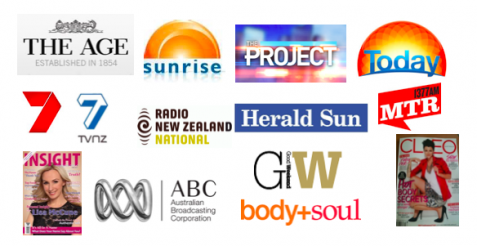The image captures a detailed layout of a variety of print and broadcast media. Prominently featured are several magazines, including titles such as "Sunrise," "Herald Sun," "Projects," "Today," and "GIW, Body+Soul." Additionally, the page showcases references to various radio channels and stations, notably including the Australian Broadcasting Corporation (ABC). A noteworthy historical detail is the established year, 1854, indicating a long-standing legacy in media history.